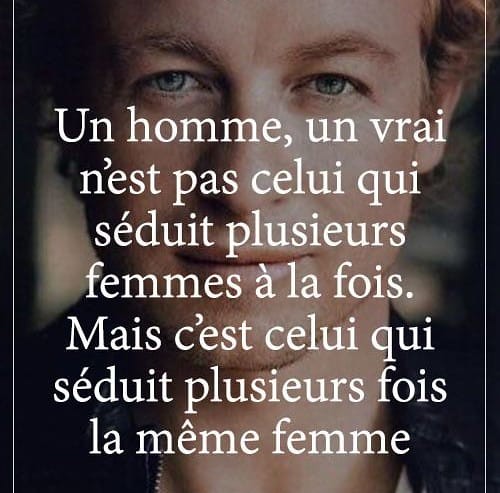The image is a vertical rectangular advertisement, likely from a magazine or an online TV screenshot, featuring a close-up of a man's face from the forehead down. The man, who is white with blue eyes and brown hair, appears to be clean-shaven and smiling, posing directly for the camera. The background is blurred with hints of white, and a black stripe runs vertically down both sides of him. He is dressed in black attire. The ad includes a significant amount of text in French, prominently displayed in white lettering across the front. Key phrases in the text include "unhom," "un-v-r-a-i," "c-e-l-u-i," "s-e-d-u-i-t," and "p-l-u-s-i-e-u-r-s," suggesting a motivational theme or message. The man’s direct gaze and upright posture further emphasize the ad’s impactful and engaging nature.